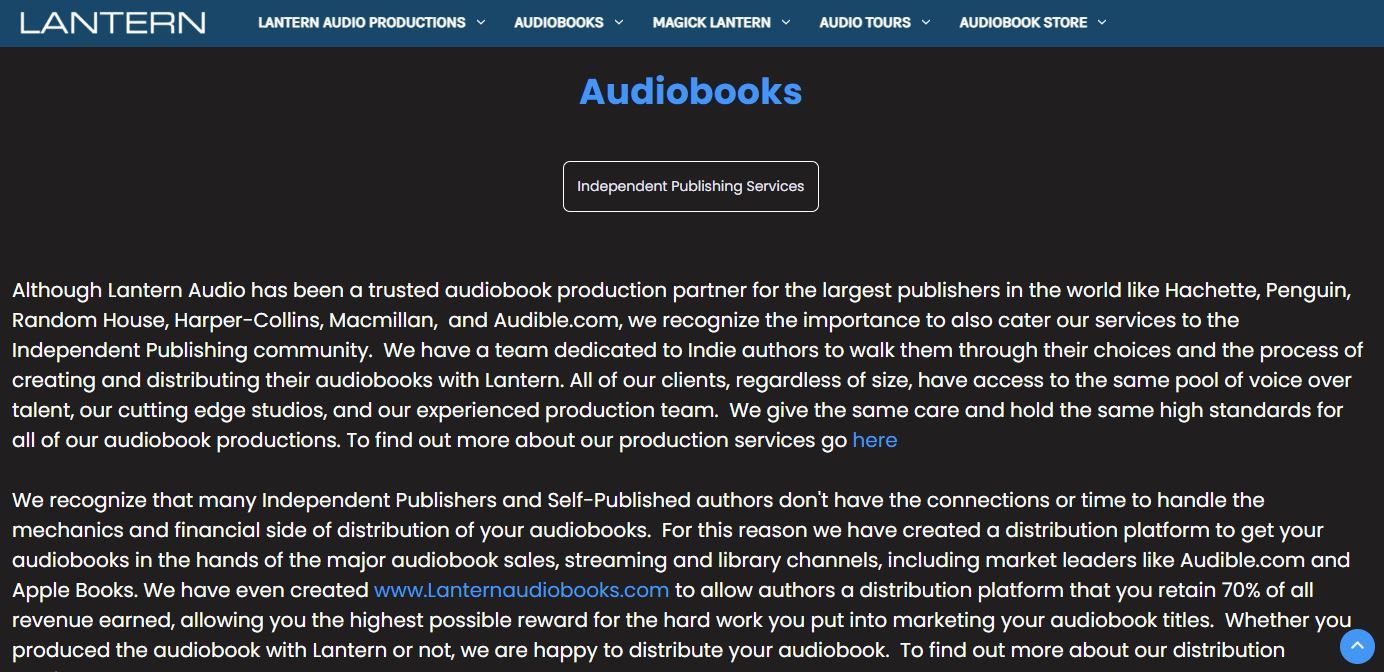### Detailed Caption for the Image:

In this screenshot, the top left corner prominently features the word "Lantern" in white letters. Adjacent to this are multiple tabs, each accompanied by a dropdown arrow. The tabs read: "Lantern Audio Productions," "Audiobooks," "Magic Lantern" (with "Magic" notably spelled with a 'K' at the end), "Audio Tours," and "Audiobook Store."

The background of the screenshot is predominantly black. In striking blue font, the word "Audiobooks" is displayed prominently on the screen. Just below this, encased in a rectangular enclosure, the phrase "Independent Publishing Services" is featured.

Two paragraphs are listed within this enclosure. The first paragraph reads:

"Although Lantern Audio has been a trusted audiobook production partner for the largest publishers in the world like Hachette, Penguin Random House, HarperCollins, Macmillan, and Audible.com, we recognize the importance of also catering our services to the independent publishing community. We have a team dedicated to indie authors to guide them through their options in the process of creating and distributing their audiobooks with Lantern. All of our clients, regardless of size, have access to the same pool of voice-over talent, our cutting-edge studios, and our experienced production team. We give the same care and uphold the same high standards for all of our audiobook productions. To find out more about our production services, go [here] (with "here" likely being a hyperlink)."

The second paragraph states:

"We recognize that many independent publishers and self-published authors don't have the connections or time to handle the mechanics and financial aspects of distributing their audiobooks. For this reason, we have developed a distribution platform to get your audiobooks into the hands of major audiobook sales, streaming, and library channels, including market leaders like Audible.com and Apple Books. We have even created www.lanternaudiobooks.com to provide authors with a distribution platform where they can retain 70% of all revenue earned, offering the highest possible reward for the hard work put into marketing audiobook titles. Whether you produce the audiobook with Lantern or not, we are happy to distribute your audiobook. To find out more about our distribution services…"